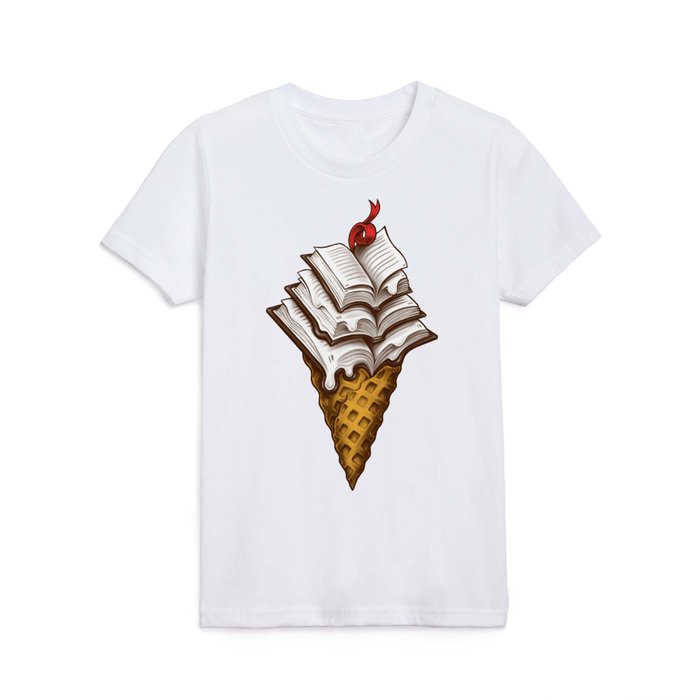This image depicts a plain white t-shirt with short sleeves and a rounded collar, laid out flat against a white background. The focal point of the t-shirt design is a whimsical, artistic depiction of a brown waffle cone. Instead of traditional ice cream scoops, the cone supports three open books stacked on top of each other, creating the illusion of melting ice cream. The pages of the books are white, while the covers are brown, and they appear to be dripping from their respective sides – with the bottom book dripping from the left, the middle book from the left, and the top book from the right. At the very top of the stack, there is a red ribbon that is artistically curled and v-cut at the top, resembling a cherry on top of an ice cream cone. The image evokes a playful contrast between knowledge and a tasty treat, suggesting an intersection of learning and indulgence.